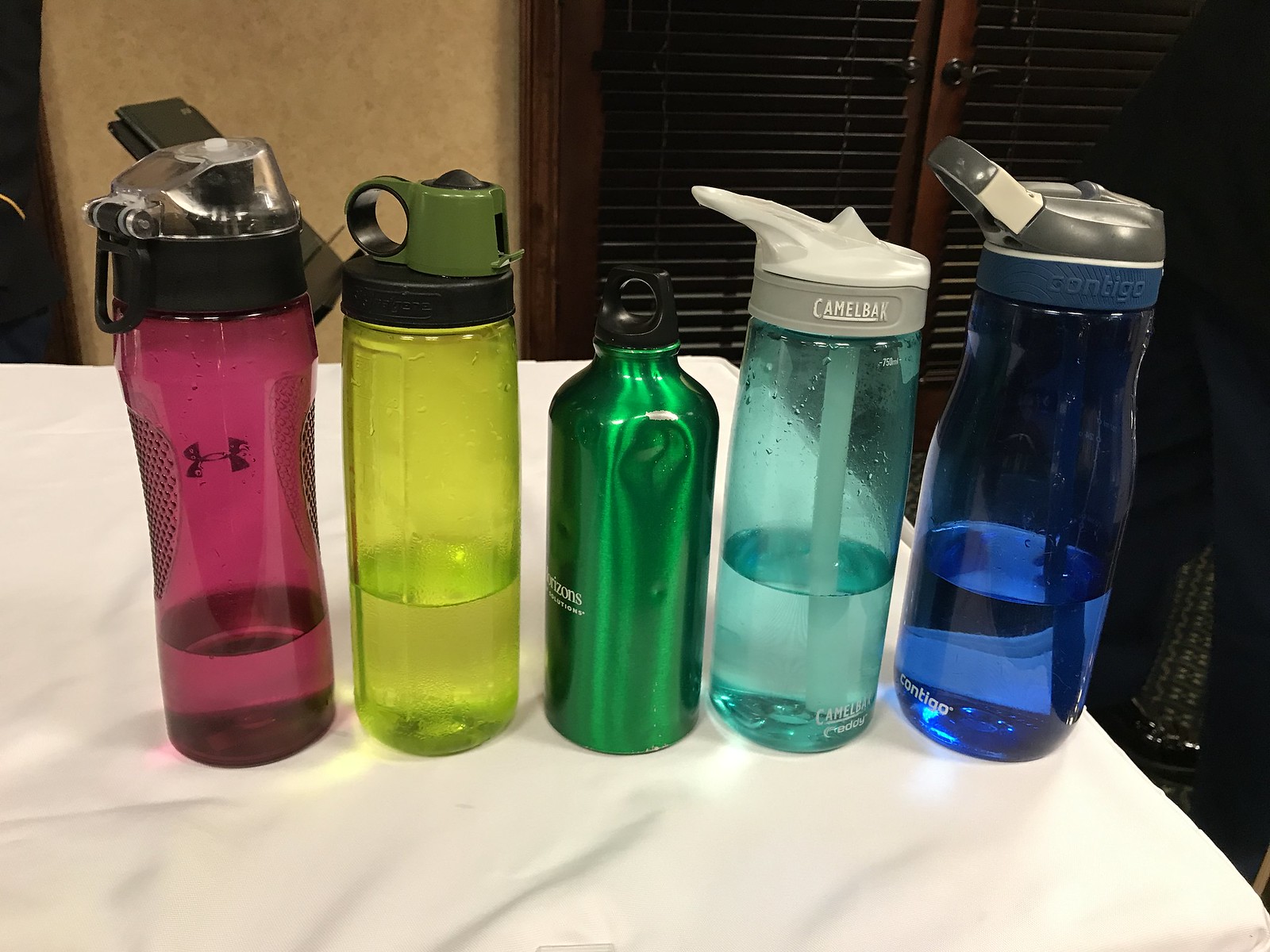The image captures a kitchen countertop viewed at an angle from the left-hand side almost all the way to the right-hand side, with a light brown wall and dark brown cabinets in the background. Five distinctive water bottles are aligned from left to right on this white, potentially marble, countertop. 

The first bottle on the left is pink and semi-transparent with a black and clear top, containing a small amount of water. The second is a translucent, fluorescent lime green bottle with a black top, also partially filled. The third bottle, situated in the middle, is a darker green aluminum canister with lighter green swirls and a black top; this one is not see-through. Moving right, the fourth bottle is light blue and translucent with a white top, visibly containing a straw and water. The final bottle on the far right is a darker blue translucent plastic with a grey top featuring a white patch, and the text "CONTIGO" in blue lettering, revealing the water level and a straw inside. In the very right of the frame is a glimpse of a man in a dark blue shirt.